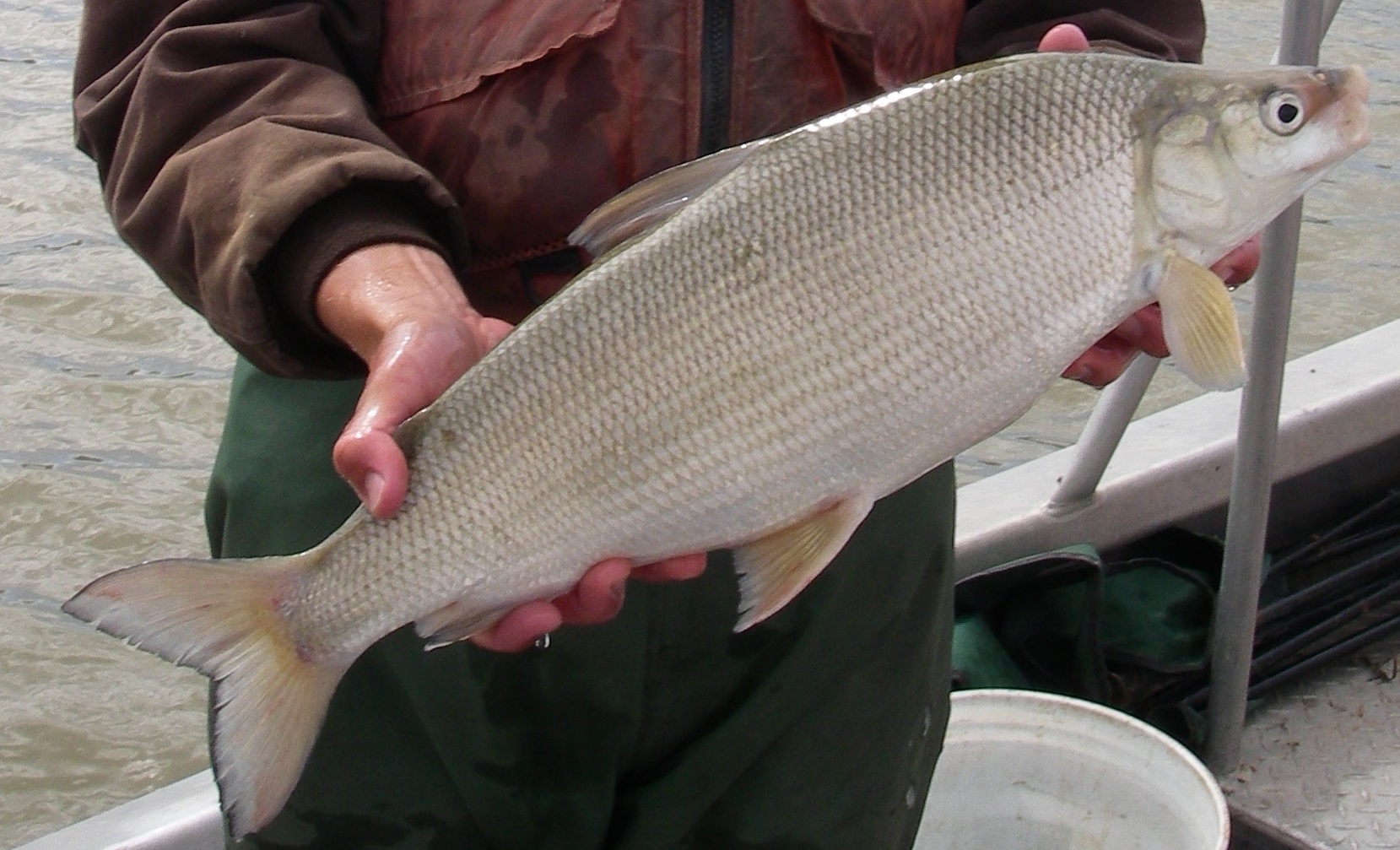This outdoor daytime photograph captures a Caucasian individual, whose gender is not clearly discernible, standing on the deck of a boat. The person is clad in a brown leather jacket, with a fishing vest over it, and green pants. They are holding a large, silver-colored fish horizontally across their body, with one hand supporting its head in the upper right-hand corner of the frame and the other gripping its tail in the lower left-hand corner. The fish, adorned with gray scales, has a black eye with a white eyebrow, prominent dorsal and belly fins, and a Y-shaped tail. 

Behind the person, there is a plastic white bucket on the deck, partially cut off by the frame, and a set of steel railings, beyond which a body of water is visible, indicating a calm day with minimal ripples. The boat's side, exhibiting shades of silver, white, and gray, forms the backdrop of the lower half of the image, while the expansive water occupies the upper half. The image has a landscape orientation, emphasizing the serene maritime setting.